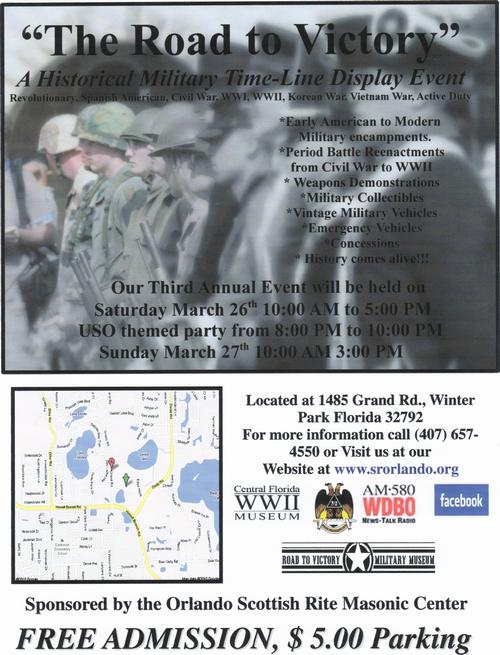The promotional piece entitled "The Road to Victory: A Historical Military Timeline Display Event" presents a comprehensive and visually engaging advertisement for a historical exhibit taking place at 1485 Grand Road, Winter Park, Florida. The top section of the piece features the event's title against a gray and black background. This section provides an overview of the historical periods covered, including the Revolutionary War, Spanish-American War, Civil War, World War I and II, Korean War, Vietnam War, and current active duty. Adjacent to this information, a list details various attractions such as early American to modern military encampments.

The central part of the advertisement showcases a black and white image of soldiers which progressively blurs towards the right, accompanied by a map on the left-hand side and additional event details on the right. The entire layout is bordered by a thin black rectangular frame, creating a clear division between sections.

Sponsors for the event include the Central Florida WWII Museum, AM580, Facebook, and Orlando Scottish Rite Masonic Center. Key information, such as the free admission with a $5 parking fee, is prominently displayed at the bottom of the advertisement in large gray letters.